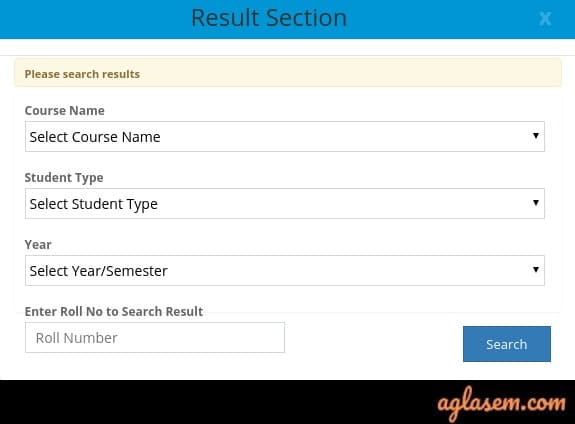This is a screenshot of an online menu interface for a results page. At the very top, there is a purple bar with the text "Results Section" written in black font. In the upper-right corner of this bar, there is a white "X" icon. Below this bar, the background is white with a beige rectangle that contains red font text stating "Please search results." 

Further down, there is a label in gray font that reads "Course Name." Underneath this label, there is a rectangular drop-down menu outlined in black, with the default text "Select Course Name" and a downward-facing arrow indicating the menu can be expanded. 

Following this, another gray font label reads "Student Type," below which is a second drop-down menu labeled "Select Student Type." Further down, a gray font label reads "Year," followed by another drop-down menu with the text "Select Year/Semester." 

Below this, the text in gray font reads "Enter Roll No to Search Results," with an adjacent rectangular input field labeled "Roll Number" in gray font. 

In the lower-right corner of the interface, there is a purple rectangle containing the text "Search" in white font. At the very bottom of the page, there is a black rectangle with the text "AGLASEM.com" written in yellow cursive font.